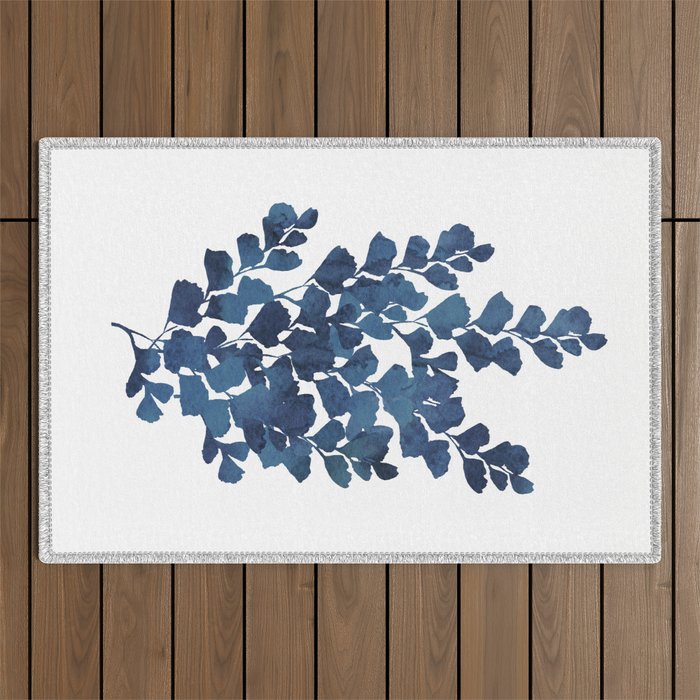The image depicts a horizontally-oriented painting with a subtle, fabric-like white background that features intricate sewing designs along the edges. The focal point of the piece is a detailed depiction of a tree branch with numerous small leaves, rendered in various shades of blue. These blue hues range from deep navy to lighter tones, with the entire piece seemingly created using watercolor techniques, giving it a soft, almost pressed-on appearance. The painting is mounted on a series of wooden slats, which comprise the wood-paneled wall, providing a rustic contrast to the artwork. The lighting is even and shadow-free, suggesting a gallery setting or professional digital display. The branch, adorned with approximately 50 to 60 finely outlined leaves, extends sideways across the canvas, capturing a sense of organic movement.